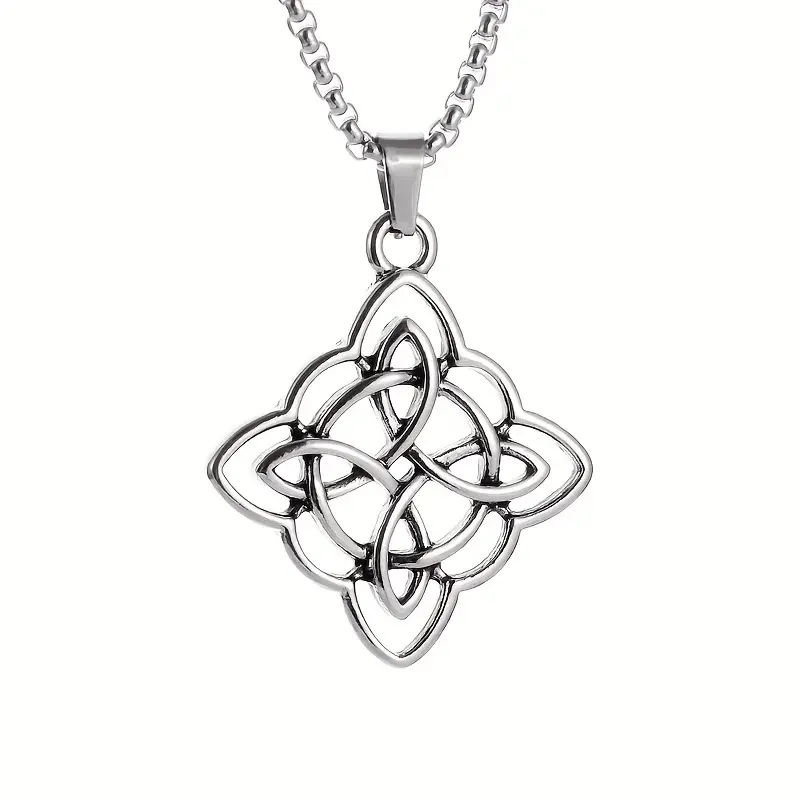The image features a close-up view of an elegant silver necklace against a white background. The necklace consists of a delicate silver chain that loops through a clasp, which dangles gracefully. Attached to the clasp is a small circular ring from which a uniquely designed pendant hangs. The pendant itself is diamond-shaped with gently curved lines at its edges, adding a touch of femininity and elegance. Inside the diamond shape, a central circular ring is adorned with teardrop shapes at the top, sides, and bottom, creating an intricate, overlapping, floral-like pattern. The background is stark white, highlighting the fine workmanship and shimmering details of the silver jewelry, which slightly tilts towards the right side of the image. Light from the right accentuates the pendant’s contours and elegant design.